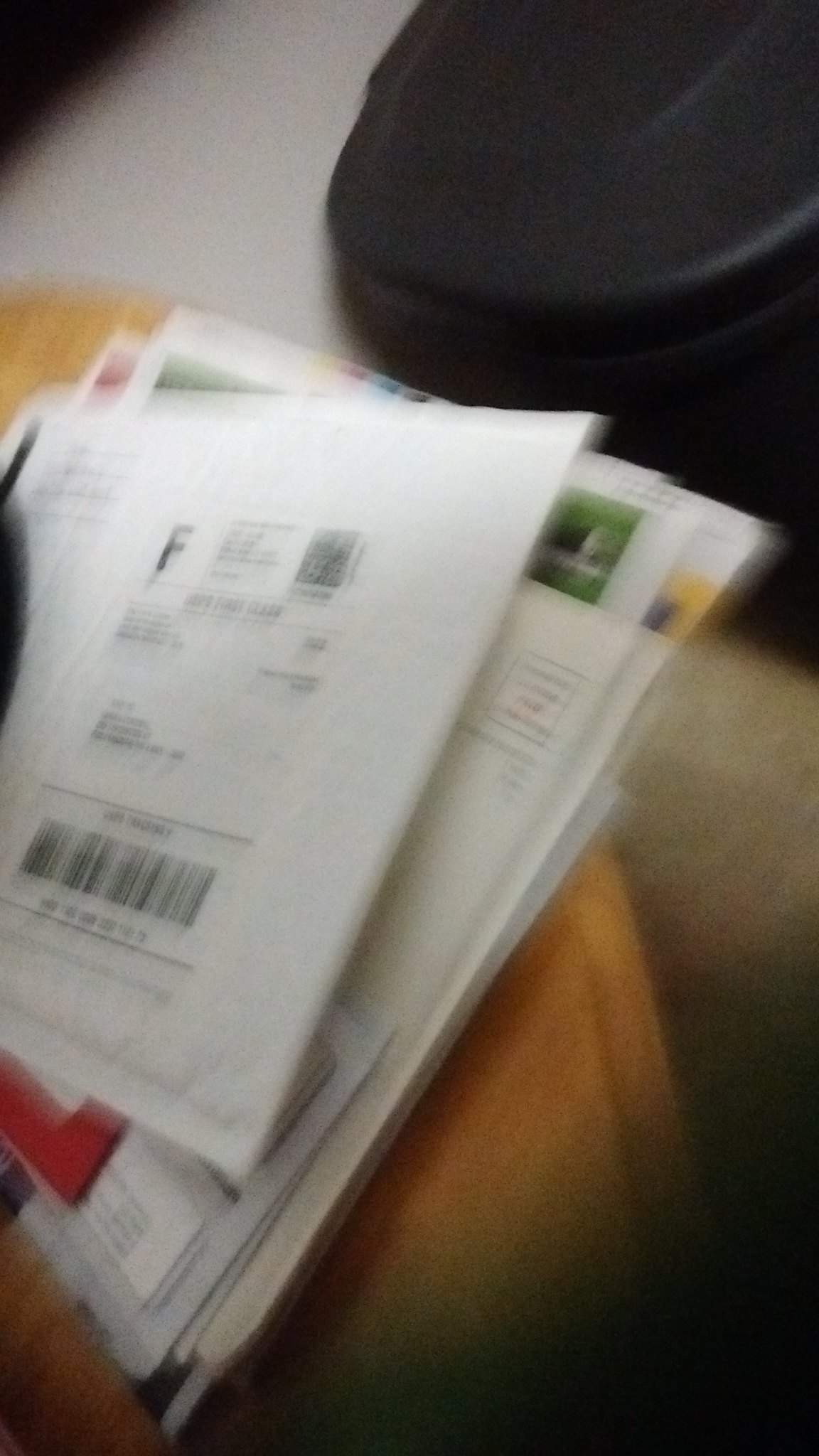A vertical indoor image captures a scattered pile of approximately seven to eight pieces of mail positioned on the left side and center of the frame. The assortment includes various types of postal items, such as parcel envelopes featuring pre-printed labels and barcodes, as well as standard letters adorned with stamps. The envelopes vary in size, with some being larger and thicker than others. The mail rests atop a fabric surface of vivid orange hue, adding a striking contrast to the scene. In the background, in the upper right-hand corner, a round black object can be seen, subtly obscured but contributing to the overall context of the setting.